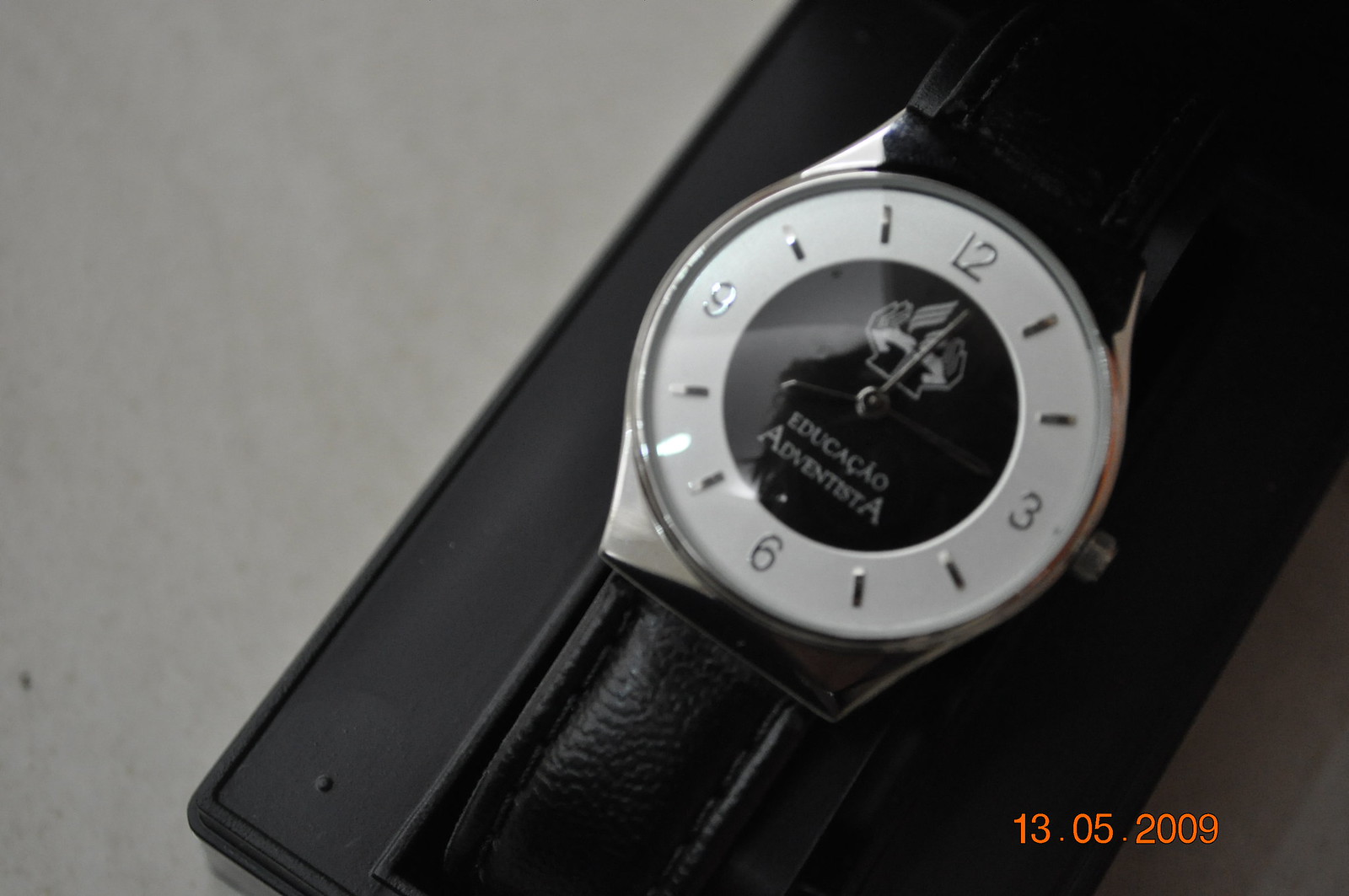A photograph dated 13.05.2009, as indicated by an orange date stamp at the bottom. The image depicts a classic wristwatch resting on a dove gray surface. The wristwatch is nestled within a sleek black box. Notably, a silver knob is visible on the side of the watch face. The watch boasts a black leather strap accented with black stitching. The clock face features a minimalist design with a white background. Prominently displayed silver numerals mark the 12, 3, 6, and 9 positions, while silver dashes denote the remaining hours. A small black circular section at the center of the clock face encloses a white icon, surrounded by dark-colored hands indicating the time. Beneath this center lies some concise white writing. The photograph captures the details of the watch clearly and crisply.